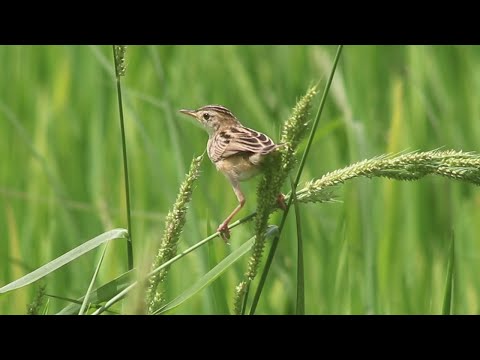In this captivating image, a small brown bird with a white underbelly is perched delicately on a bent wheat stalk. The bird exhibits intricate patterns of black and brown horizontal lines on its wings and head, accentuating its detailed plumage. Its black eyes are intently focused to the left, and it stands with extended legs gripping the stalk lightly, reflecting its minimal weight. The surrounding environment is lush with green, blurred tall grass or wheat, and other stems with furry leaves, enhancing the scene's serene, springtime ambiance. The overall composition, featuring dominant earthy browns and vibrant greens, creates a peaceful and natural tableau, perfect for depicting the innocence and lightness of this keenly observant bird.